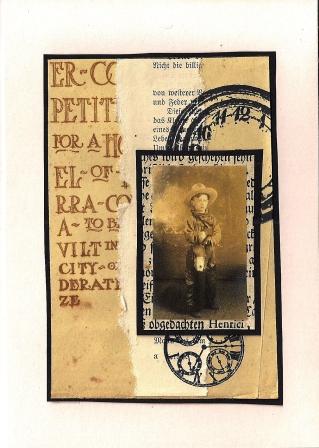The image appears to be a vintage-style piece of artwork resembling a book cover or a postcard, set against what looks like aged, overlapping excerpts from various texts, possibly in a foreign language like French. Domineering the background is an old, textured piece of paper, cluttered with cropped, indistinguishable text fragments. Layered over this, there's an intricate arrangement of elements: in the top part, a partially cut-off clock face labeled 1 through 12, and at the bottom, the intricate gear mechanisms of a watch. Central to the composition, slightly right of center, is an old, black-and-white photograph of a young boy, likely around five years old, posed in a full cowboy outfit complete with a hat, jacket, jeans, and boots. This photo, bordered by a dark rectangle, is superimposed over the textured background, giving the impression of a scanned or printed image on a white piece of paper. The entire composition invokes a nostalgic, layered aesthetic evocative of old newspapers or postcards.